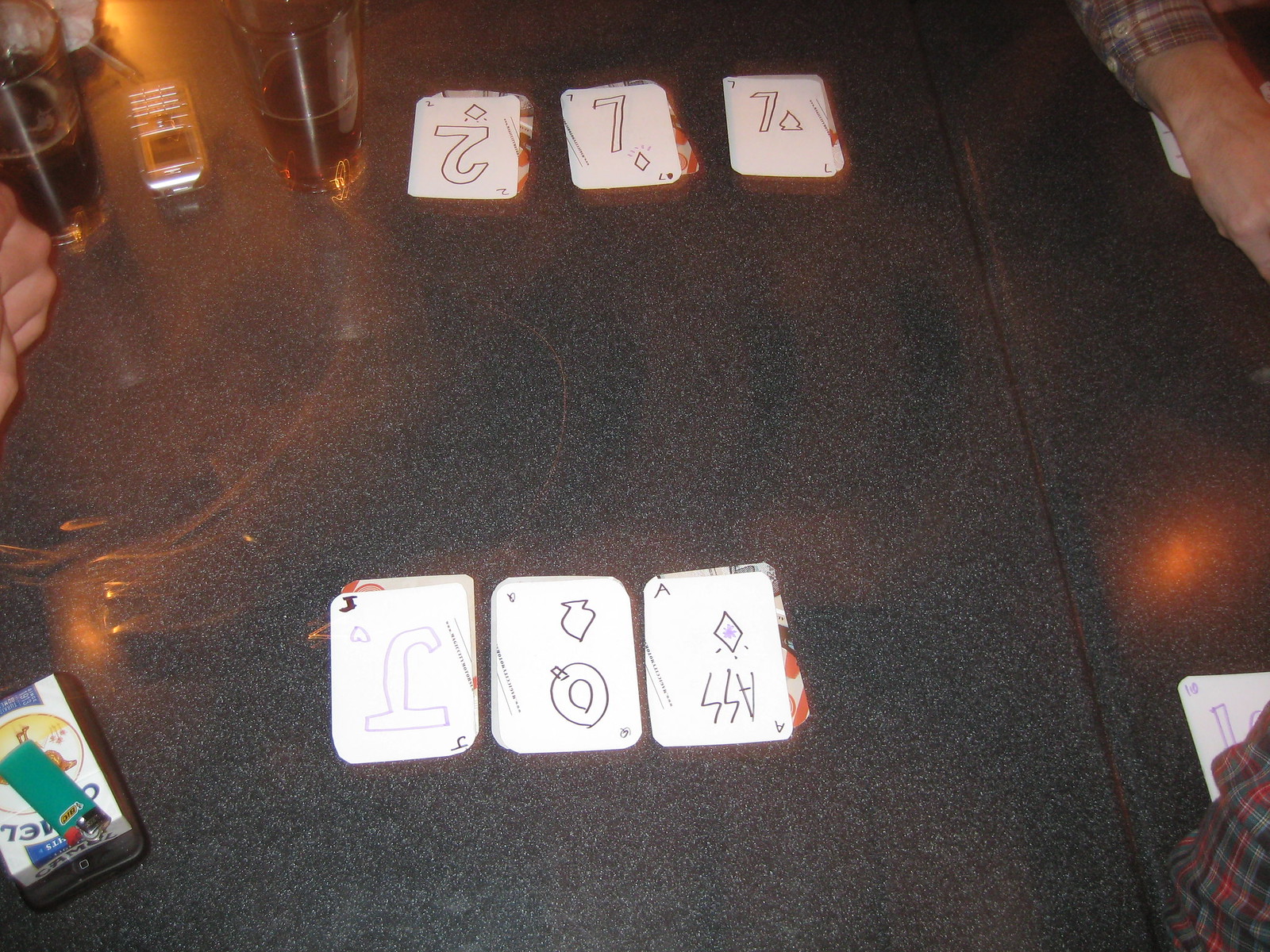In this indoor photograph, likely taken at a restaurant or bar, two individuals are engaged in a card game using handmade cards. The table is adorned with three stacks of intricately designed cards, rendered in pen and ink, laid out on either side. In the bottom left corner, a pack of Camel cigarettes is topped with a distinctive green Bic lighter. Partially within the frame in the bottom right, the edge of a red and green flannel sleeve hints at the presence of one of the participants. To the upper left, two tall glasses, one containing a medium brown liquid and the other a darker brown, sit closely with a cell phone positioned between them. The tabletop itself has a distinctive black and white speckled pattern. An orange light source casts a warm glow across the scene from the upper left, while a portion of a hand, likely belonging to a Caucasian male based on the partial view of his shirt, is visible in the upper right. The overall ambiance suggests a casual and relaxed atmosphere as they enjoy their drinks and game.